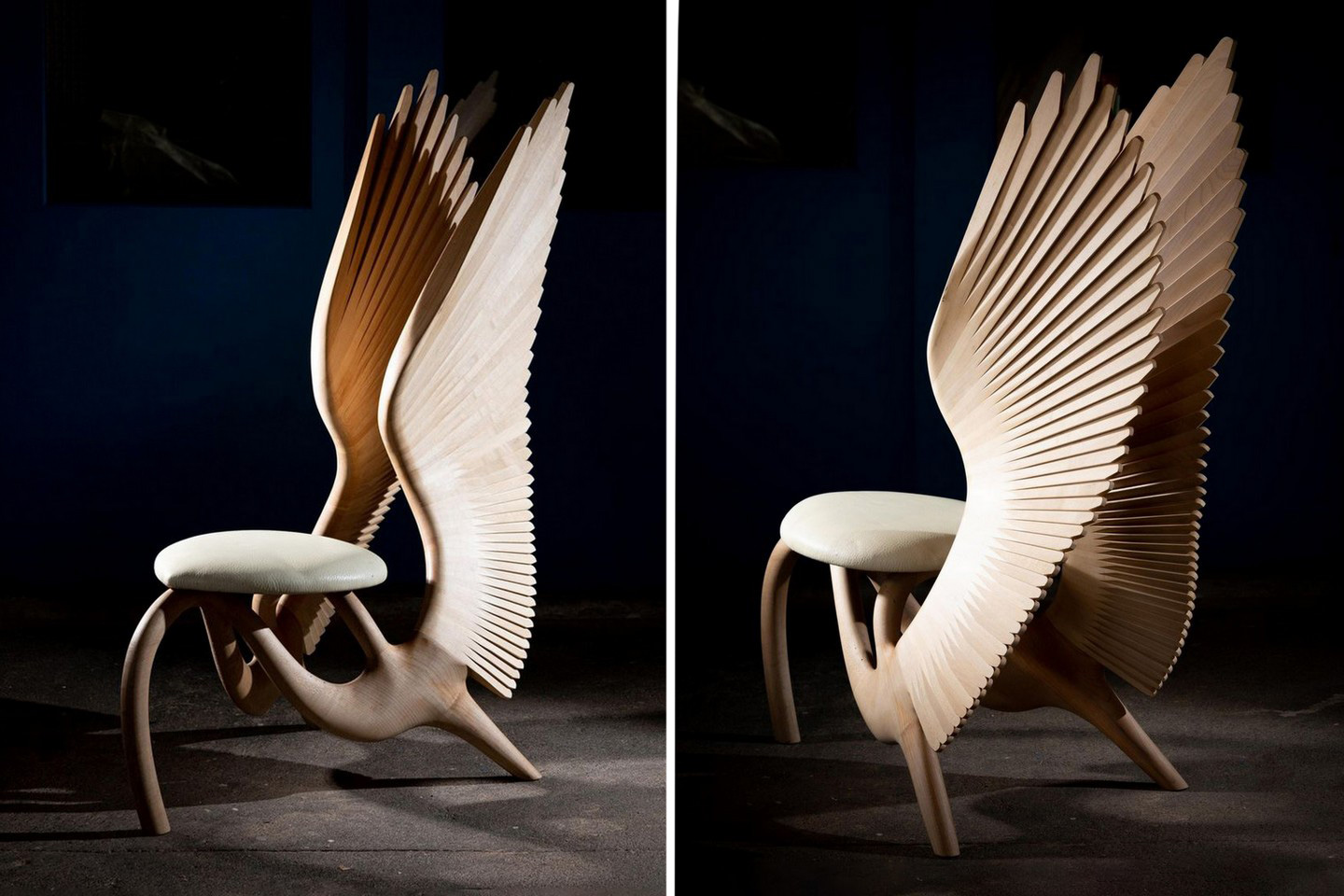The image showcases two side-by-side perspectives of an innovative, bird-inspired chair sculpture set against a black backdrop with a gray, possibly concrete surface. The seat is circular, with a light, greenish eggshell color that appears almost leather-like. The chair is supported by three legs. The front leg, crafted from a curved piece of wood, resembles a beak-like structure. The most striking feature of the chair is the pair of expansive, angelic wings that emerge from the back, creating the rear two legs. These wings, intricately detailed with numerous feather-like patterns, are white on the outside and gradate from light to dark brown on the inside. The left image provides a side view, while the right image offers a back view, reinforcing the chair's artistic and functional design. The juxtaposition of the two angles emphasizes the chair's creative form, blending aesthetics with utility.